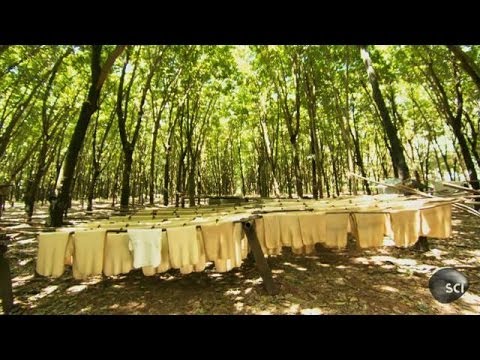The image appears to be a screenshot from a TV show or movie, identifiable by the thick black bars at the top and bottom (letterboxing) and a circle with the text "SCI" in the bottom right, which could be a network logo. The perspective is low to the ground, around two feet high, offering a striking view of a dense forest. The forest is filled with tall, slender trees whose trunks stretch upward, disappearing into the leafy canopy that blocks out the sky. Sunlight filters gently through the leaves, casting dappled light onto the scene below.

The forest floor is mostly covered in brown grass or dirt, and prominently features numerous rows of objects that resemble either fabric or animal skins hanging on clotheslines. These items vary in color from white to possibly yellow or orange. They are arranged in multiple rows, with each row containing several pieces, creating an almost infinite visual depth as they recede into the background. The items are neatly displayed, suggesting some form of methodical arrangement. The overall image captures the intricate patterns and immense scale of both the forest and the hanging objects, creating a captivating and mysterious atmosphere.